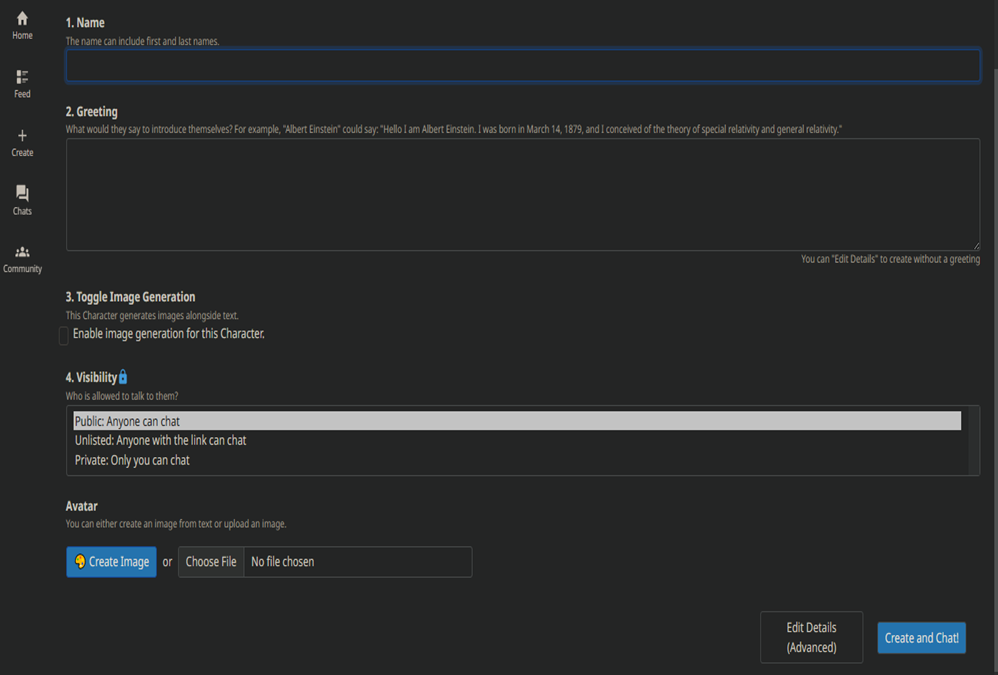The image displays a web page with a sleek black background, accented predominantly in shades of black, white, and blue, with minor touches of yellow. The left-side vertical panel features a navigation menu, listing options with corresponding icons: 'Home' with a house icon, 'Feed,' 'Create' with a plus icon, 'Chats' with a chat bubble icon, and 'Community' with profile heads.

At the top center section is a step-by-step form labeled with numbers. 

1. **Name**: This section highlights a long rectangular box outlined in blue where users are instructed to enter names, specifying that both first and last names are acceptable.
   
2. **Greeting**: Users are prompted to provide an introductory greeting. An example is displayed, where "Albert Einstein" might write: "Hello, I'm Albert Einstein. I was born on March 14, 1879, and I conceived the theories of special relativity and general relativity." Below this example is a blank rectangular box for users to input their own greetings. Additional text at the bottom indicates that users can edit details to proceed without a greeting if preferred.
   
3. **Toggle Image Generation**: This section involves a feature that enables image generation alongside text for the specified character. A checkbox allows users to enable or disable this function.
   
4. **Visibility**: Marked with a blue lock icon, this section dictates the privacy and visibility settings for the character being created.

At the very bottom of the image, there is an unrelated promotional message: "Go to Beadaholique.com for all of your beading supplies needs!"